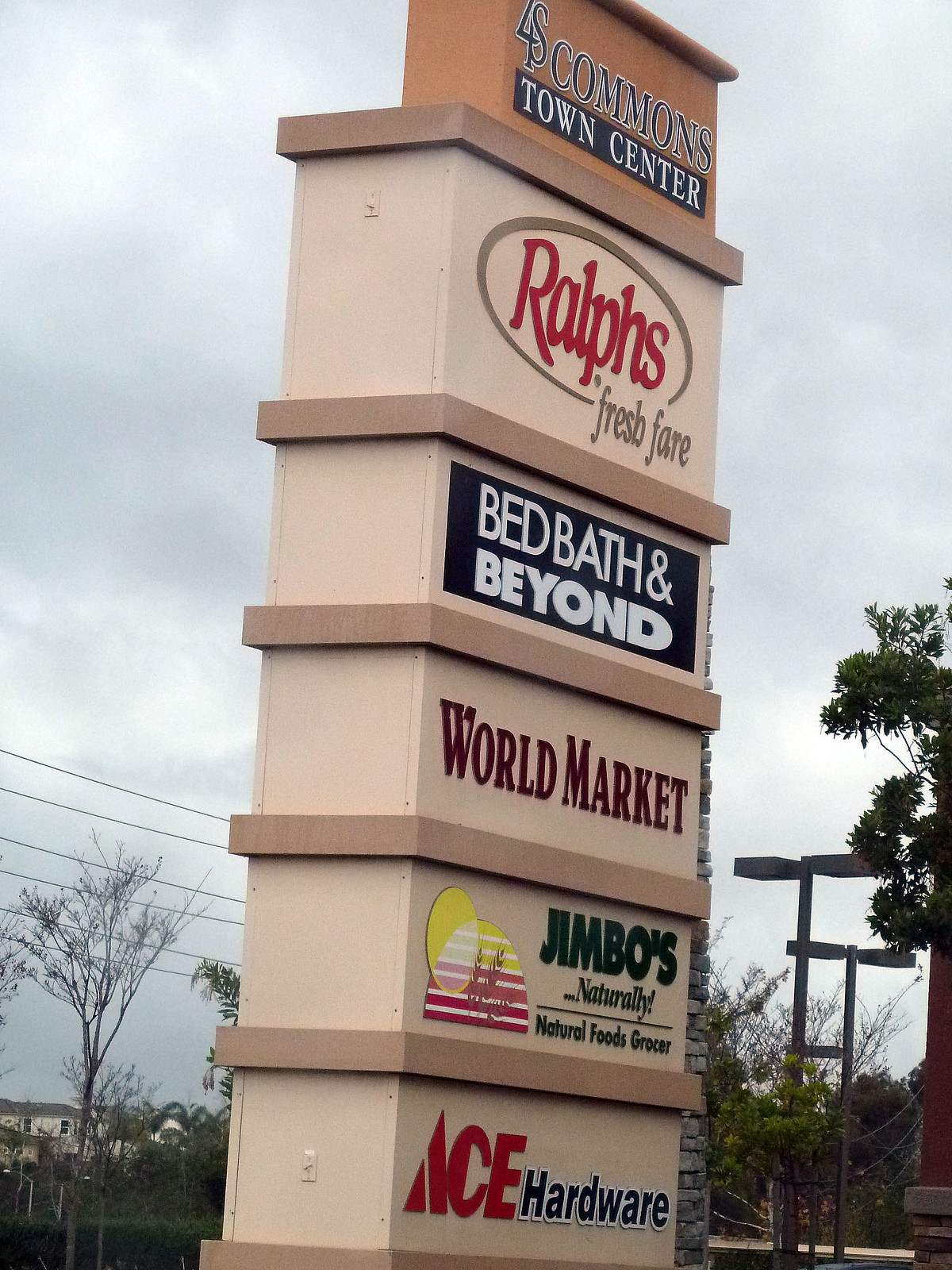The photograph captures a tall, beige-colored column sign for a strip mall, prominently displaying the names of various businesses from top to bottom. At the very top of the sign, in large font, is "Commons Town Center," followed by "Ralph's Fresh Fare" in red letters, with the recognizable Ralph’s logo. Below Ralph's is "Bed Bath & Beyond," then "World Market," also in red letters. Continuing downward, "Jimbo's Naturally," a natural foods grocery, and finally, "Ace Hardware" are listed. The background of the image shows an overcast, cloudy sky with visible power poles and black metal streetlights. Some stonework is visible behind the sign, along with housing structures that seem to belong to a nearby subdivision nestled behind the trees. The sign itself features a color palette of tan, brown, black, white, red, burgundy, green, and yellow.